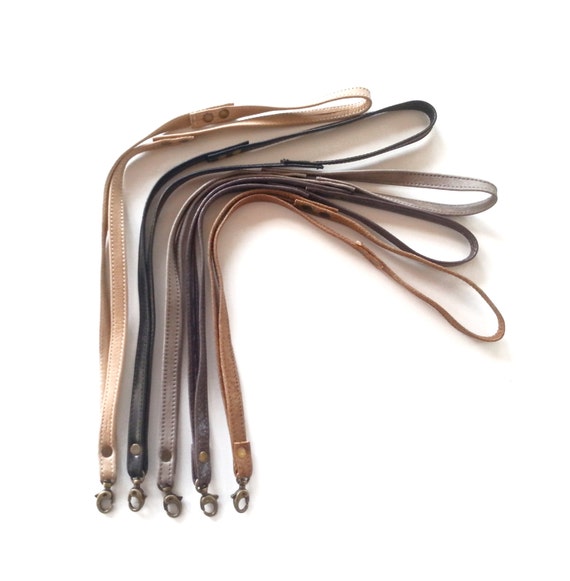The image displays five leather straps arranged side by side, each featuring a metal clasp at their bottom end. From left to right, the straps are colored beige, black, light gray, dark gray, and tan brown. The bottom of the image shows a metal pin securing the clasp in place. The straps are looped, forming a right angle toward the right side of the image where clips hold them in place. The loops are relatively closed, resembling handholds or lanyards, and the arrangement at the top is folded inward to fit within the frame.